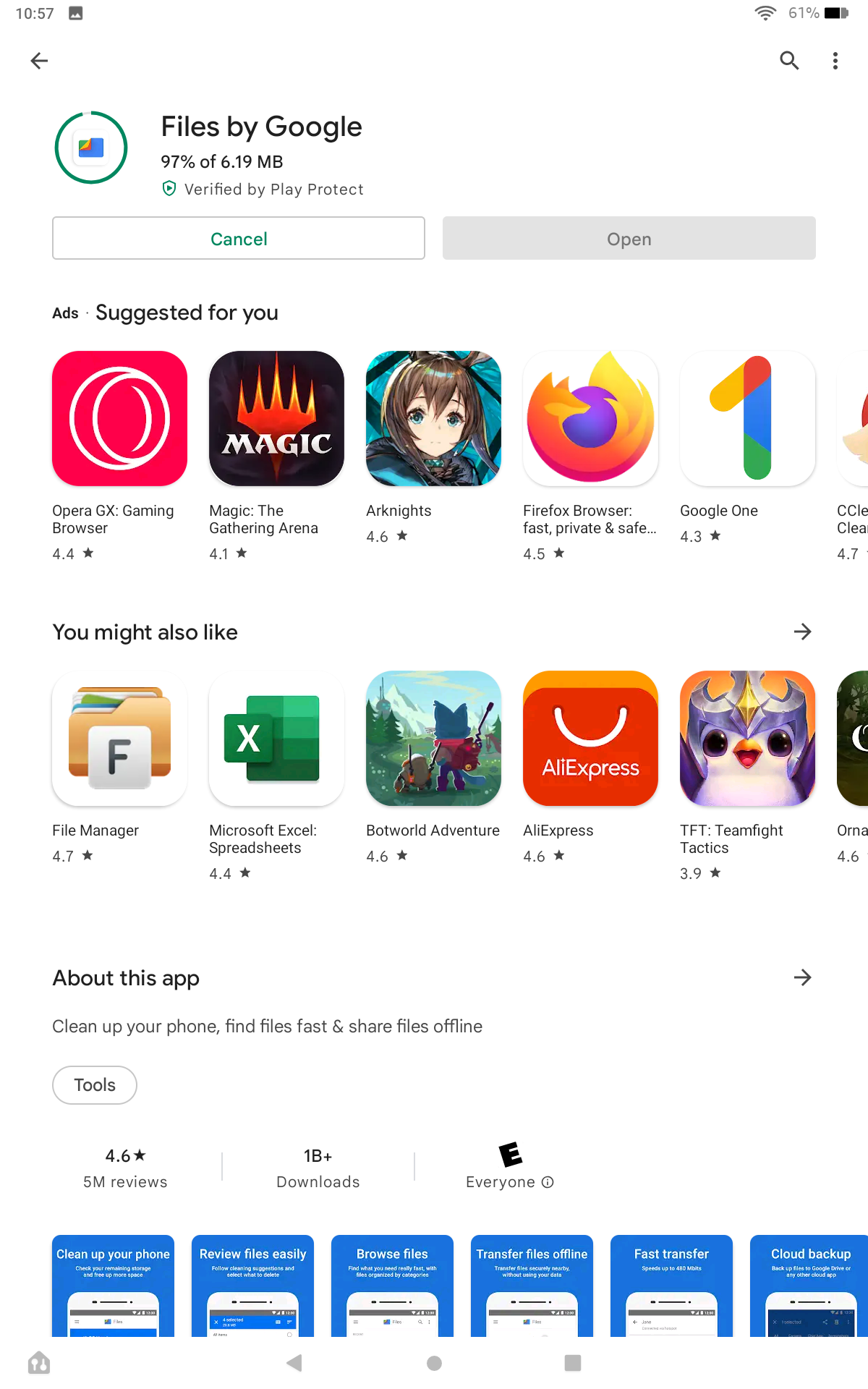The image depicts a screen detailing the download process and app suggestions from Google Play Store. The primary focus is on a nearly completed download of a file, with "97% of 6.9 MB" verified by Play Protect. Below this progress bar are two buttons: "Cancel" and "Open."

Beneath the download status, the screen features a section titled "Ads Suggested For You," listing several apps including Opera GX Gaming Browser, Magic: The Gathering Arena, Arknights, Firefox Browser, and Google One, though one app is partially obscured.

Another section labeled "You Might Also Like" offers app suggestions like File Manager, Microsoft Excel Spreadsheets, Botworld Adventure, AliExpress, TFT: Teamfight Tactics, and Doodoo Doonga. An arrow points to the right, indicating more options available.

Following this, there's a brief description headed "About This App," accompanied by another right-pointing arrow. The description reads "Clean up your phone and find files fast and share files online." Below this, the "Tools" button is prominently displayed.

The app has earned a rating of 4.6 stars from 5 million reviews and boasts over 1 billion downloads. It is rated E for Everyone. Accompanying this information is a gallery of promotional images showing various features of the app, such as "Clean Up Your Phone," "Review Files," "Easily Browse Files," "Transfer Files Offline," "Fast Transfer," and "Cloud Backup." These images appear slightly cropped, each displaying a phone demonstrating the respective feature.

In the top-left corner of the screen, the current time is shown as 10:57, while the top-right corner indicates a 61% battery level. There is also a magnifying glass icon in the top-right corner, suggesting a search function. The background of the screen is predominantly white, providing a clean and uncluttered interface.